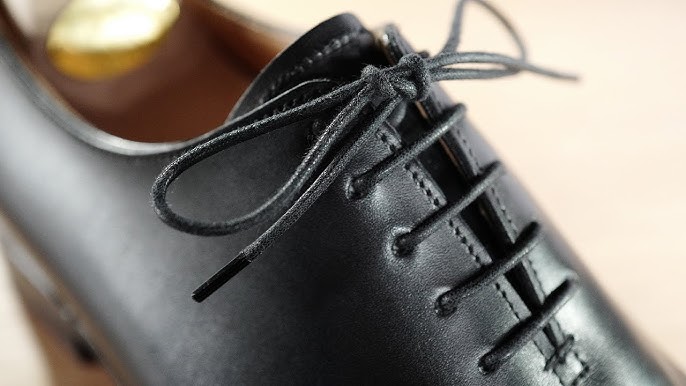This image is a close-up of a men's black leather dress shoe. The shoe features a thin, round black shoelace threaded through all the eyelets and tied in a bow near the tongue. The image highlights the central section of the shoe, providing a detailed view of the lacing and V-shaped opening. The interior of the shoe is visible near the tongue and appears to be tan or golden brown in color. The shoe has a slightly raised heel, and the background of the image is a light peach color. The photo focuses on the upper part of the shoe, excluding the toe and full back portion, and captures the stitching detail around the lace area.